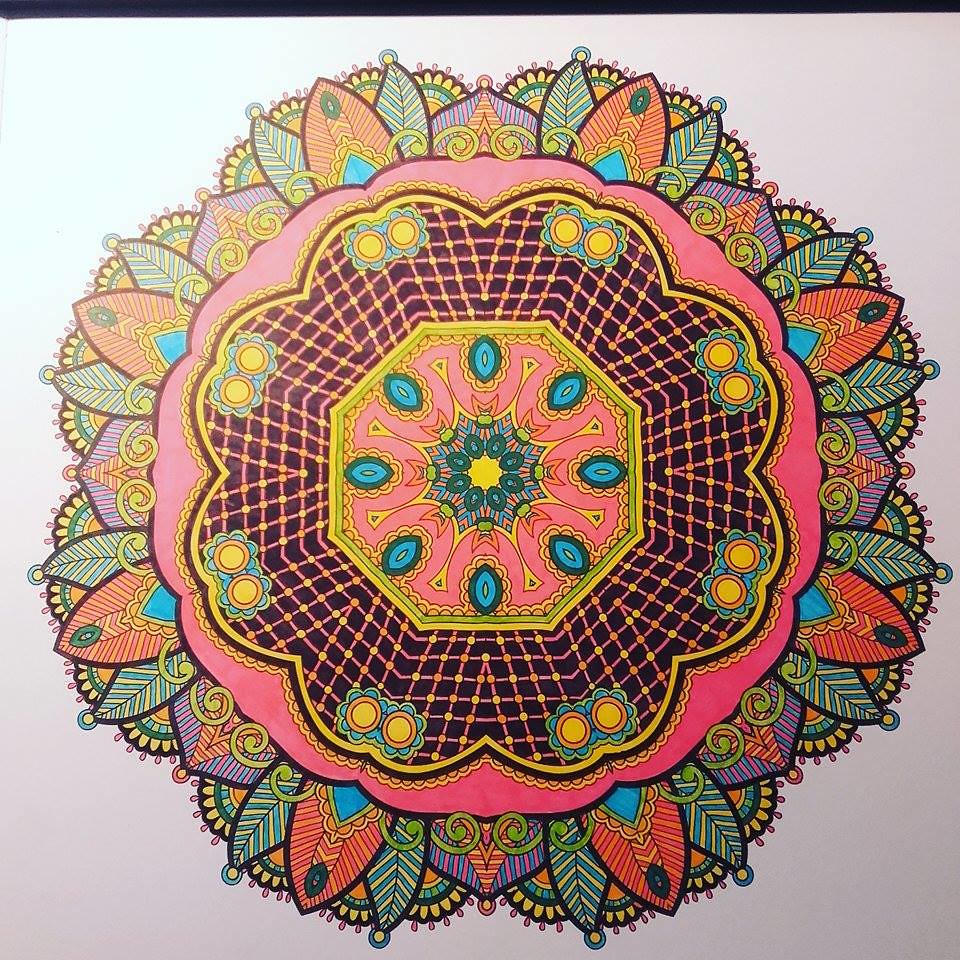The image is an intricate illustration of a mandala, set against a gradient background that transitions from light blue in the top left corner to light purple on the right-hand side. At its core, the mandala features an octagon with a yellow border and a pink interior. Surrounding the octagon, blue and green shapes dynamically float, adding to the rich tapestry of colors. This central structure is enveloped by a larger, clover-like shape, also outlined in yellow but filled with pink lines that contrast against the purplish paper.

Radiating from this clover-like form is a ring of leaves or feather-like shapes, alternating in vibrant colors of red, green, and orange, creating a warm and cool color harmony. These leaves, detailed with central lines from which colors branch out, contribute to the kaleidoscope effect that defines the mandala. The larger structure can be likened to a chrysanthemum, with pink petals that enhance the floral aesthetic.

This artwork occupies nearly the entire image, presented within a square format with a white background. An ornate circle design, it features various geometric patterns and layers that radiate outward, mimicking the style of a kaleidoscope. The top of the image is bordered by a narrow black strip, creating a contrast that draws focus to the central, multi-colored mandala.